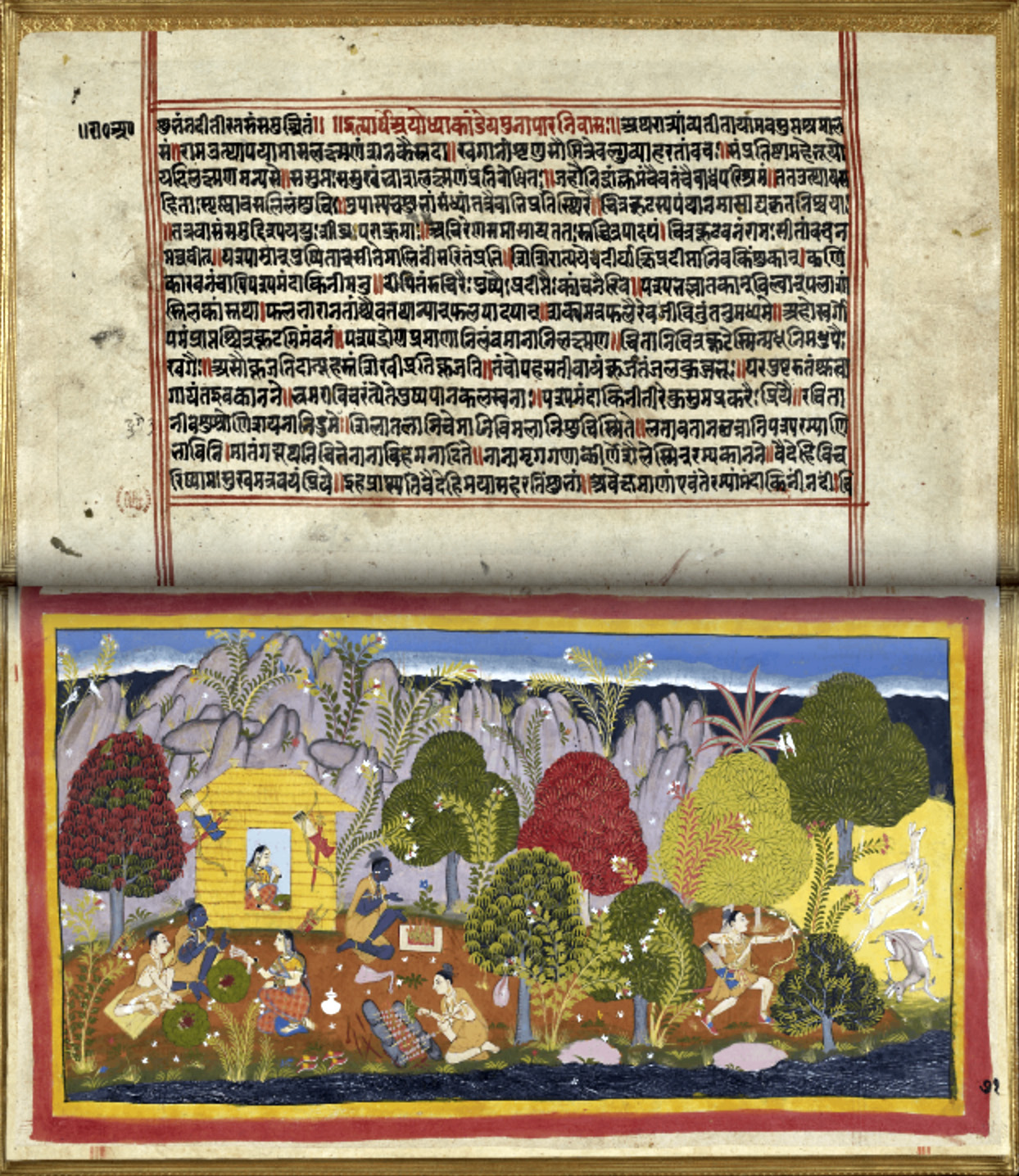This image is composed of two distinct sections. The top section contains a script that appears to be in an ancient Middle Eastern language, likely resembling Arabic calligraphy. The script is written predominantly in black ink, with a single sentence highlighted in bright red. The background of this section is a parchment-like beige, giving it an aged appearance.

The bottom section is an elaborate, stylized painting with a diverse array of elements. A variety of vibrantly colored trees—ranging from red and green to blue and light green—populate the scene. Among these trees, a group of people is depicted in various activities: three individuals are conversing on the ground, one is preparing a pack, and another is planting a tree. There is also a small yellow house nestled within the trees, housing a solitary figure gazing out of the window.

Surrounding these elements, additional details include blue water and brown ground, with gray mountains in the backdrop and a clear blue sky above. The scene is encased with yellow and red borders, enhancing its intricate, almost surreal quality. Overall, this richly detailed image combines ancient script and stylized painting to create a cohesive, visually compelling piece on parchment.